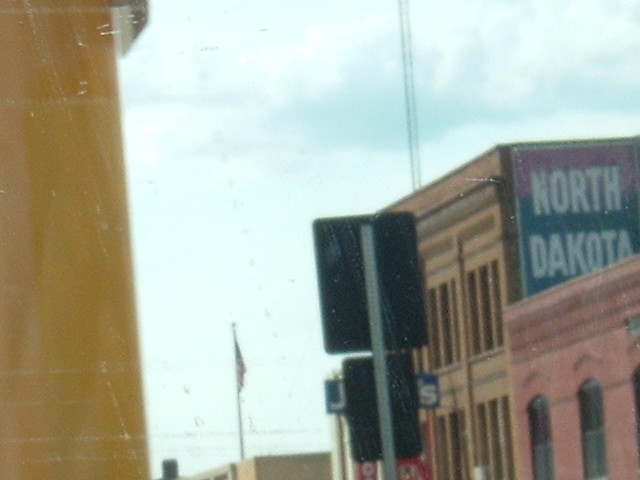This daytime landscape-oriented color photograph captures an outdoor street scene in the United States, viewed through a glass pane streaked with scratches and dirt. Prominently positioned on the right side is a tall brown building adorned with a large billboard featuring a red and blue background with "North Dakota" written in white text. Adjacent to this structure is a slightly shorter, flat-topped red building, both having multiple windows. In the center foreground, there is a silver pole with two rectangular black signs whose fronts face away from the viewer, obscuring additional details. To the left, a distant building features an American flag, distinguishable by its blue triangle and red and white stripes, hanging limply against the flagpole. Overhead, a sky adorned with clouds stretches across the background, and a yellow object is noticeable in the upper left part of the image. The overall scene is slightly blurry, reinforcing the impression of viewing through a pane of glass.